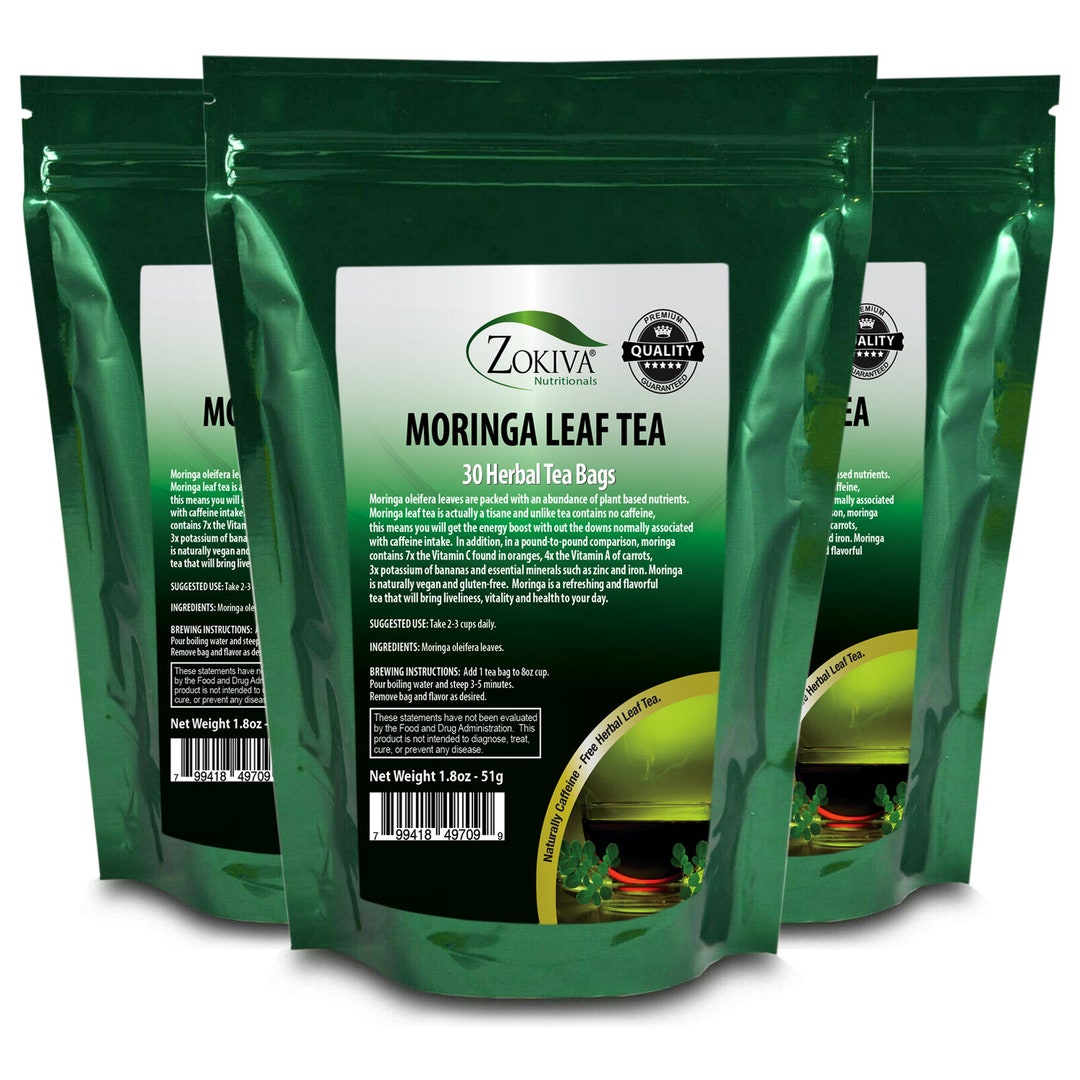The image displays three shimmering green, metallic sack-style bags of herbal tea, with one prominently in the center and two slightly obscured behind it. Each bag, adorned with a top-front seal zipper, features the label "Zokiva Nutritionals." Highlighted at the top is a premium quality stamp with a five-star guarantee. The central bag clearly reads "Moringa Leaf Tea, 30 Herbal Tea Bags," followed by detailed information on suggested use, ingredients, and brewing instructions. Descriptive text emphasizes the refreshing and nutrient-rich qualities of the tea, promising to bring liveliness and vitality. Additionally, a small picture of plants, likely the source of the tea leaves, sits in the bottom right corner along with a barcode and the net weight of 1.8 ounces (51 grams).